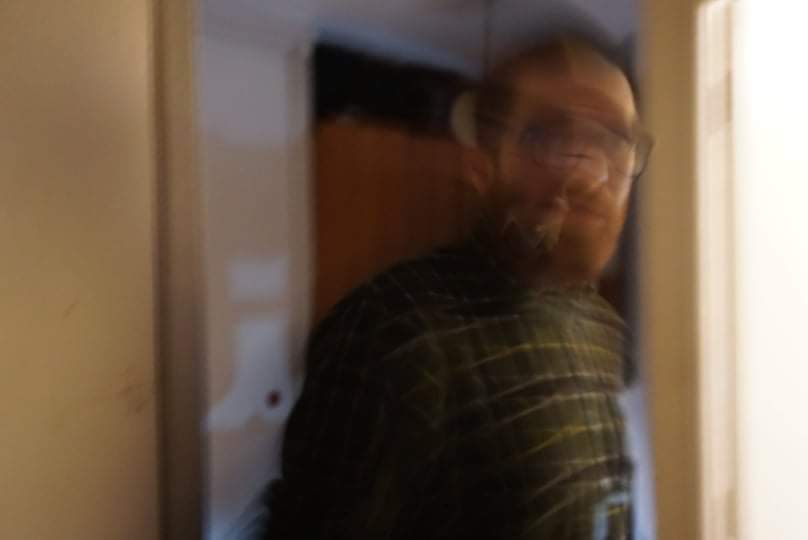In this grainy and blurred photograph, a man with a brown beard, mustache, and brown hair is captured from the chest up, positioned on the right side of the image. He appears to be in his 30s, 40s, or 50s and has slight sideburns. The man is wearing a green and yellow plaid button-down shirt with a collar. The background features tan walls and an open doorway, while to the left of the frame is a structure that could be either a corner of the wall or a wooden beam. The poor quality of the image makes it difficult to discern finer details.